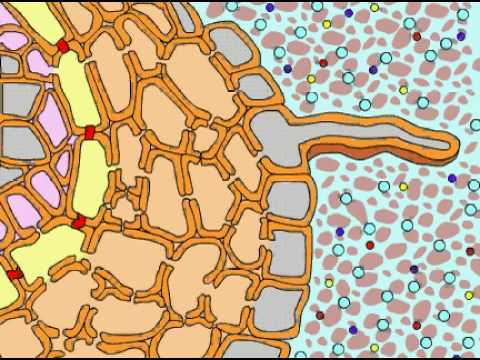The image appears to be a detailed computer diagram depicting a series of cellular structures and components. On the far right, the background is mint green, filled with numerous light blue dots, alongside darker mint green, yellow, purple, and some pinkish rock-shaped elements. Moving leftwards, there is a prominent section featuring red blood cells and small red blocks dispersed within white space, interspersed with a variety of light blue, dark blue, red, and yellow circles. This section connects to an intricate cell block arrangement outlined in orange. The cells themselves exhibit complex layering: the first layer is gray with thin orange outlines, some cells having middle portions that extend outward resembling tentacles. Following this, there is another light orange section with dark orange outlines, then a yellow layer with interspersed red blocks, a subsequent purple layer, and an innermost layer that is gray. The insides of these cellular shapes range from light sherbet orange to gray. Overall, the diagram intricately portrays cellular diversity and complexity, with repetitive detailed descriptions of multiple layers and scattered colorful elements between outlined cell walls.